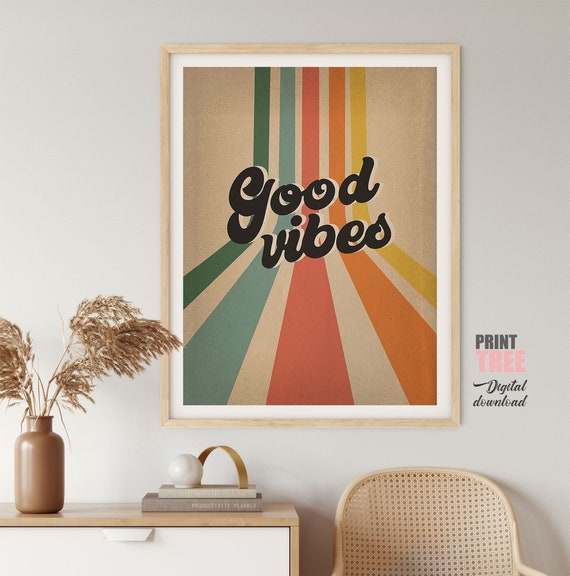The image is a realistic photograph featuring a cozy interior room. The background is a very light beige, almost off-white wall. Centrally mounted on the wall is a framed print with a light wooden frame and a white border. The print itself has a light brown or beige background with vertical stripes in green, blue, red, orange, and yellow, tapering from the top to the bottom. Across the middle of the print, in bold black font, it reads "Good Vibes." 

To the bottom left of the image is a small, stylish end table made of a light wooden frame with a white drawer. On top of this table is a brown, bottle-shaped vase filled with some dried brown plants or grass. There are also a few books on the table, topped with a white marble globe and a small golden arch decoration. 

On the bottom right side of the image is a light brown wicker chair, which adds a touch of natural texture to the space. To the right of the print, there is text in varying fonts and colors that reads "Print Tree Digital Download." The careful arrangement of these elements creates a harmonious and inviting interior.